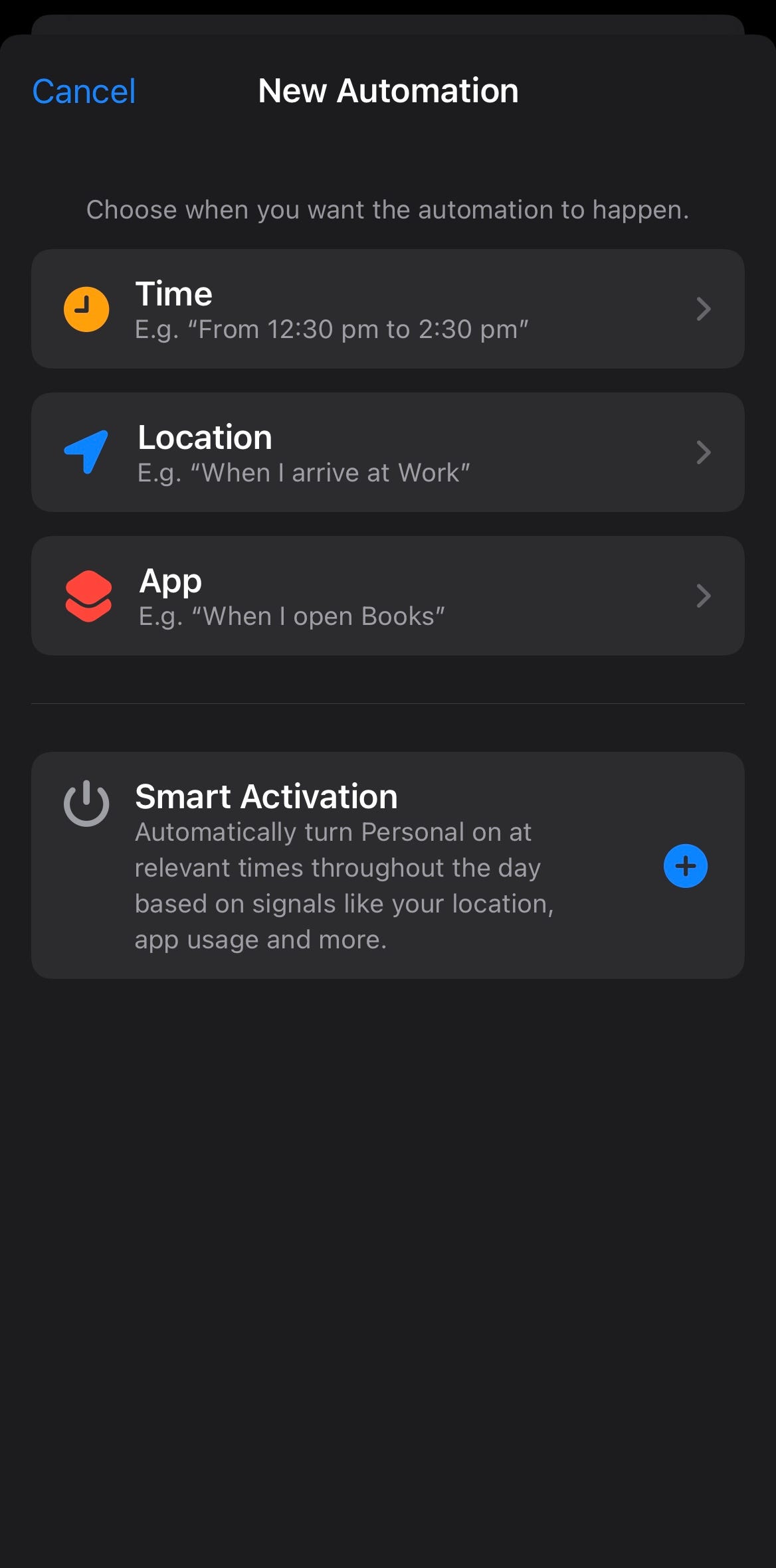The image showcases a screenshot of a cell phone screen displaying the "New Automation" settings. In the top left corner, the blue text reads "Cancel," while to its right, in white, it says "New Automation." Below this heading is a small gray sentence that instructs, "Choose when you want the automation to happen."

Three options are presented beneath this instruction, each encased in gray rectangles. The first option, labeled "Time," features an orange clock icon and includes an example, "e.g., from 12:30 p.m. to 2:30 p.m." The second option is "Location," indicated by a blue arrow pointing diagonally to the right, with an example, "e.g., when I arrive at work." The third option, "App," is marked by two red square icons stacked on top of each other, with an example, "e.g., when I open Books."

Lower in the screen, there is a gray rectangle featuring an option titled "Smart Activation," accompanied by a power button icon on its left. This setting is described as "Automatically turn personal on at relevant times throughout the day based on signals like your location, app usage, and more." To the right of this description, a blue circle with a plus sign is visible.

The remainder of the background in the image is black, giving a stark contrast that highlights the elements on the screen.